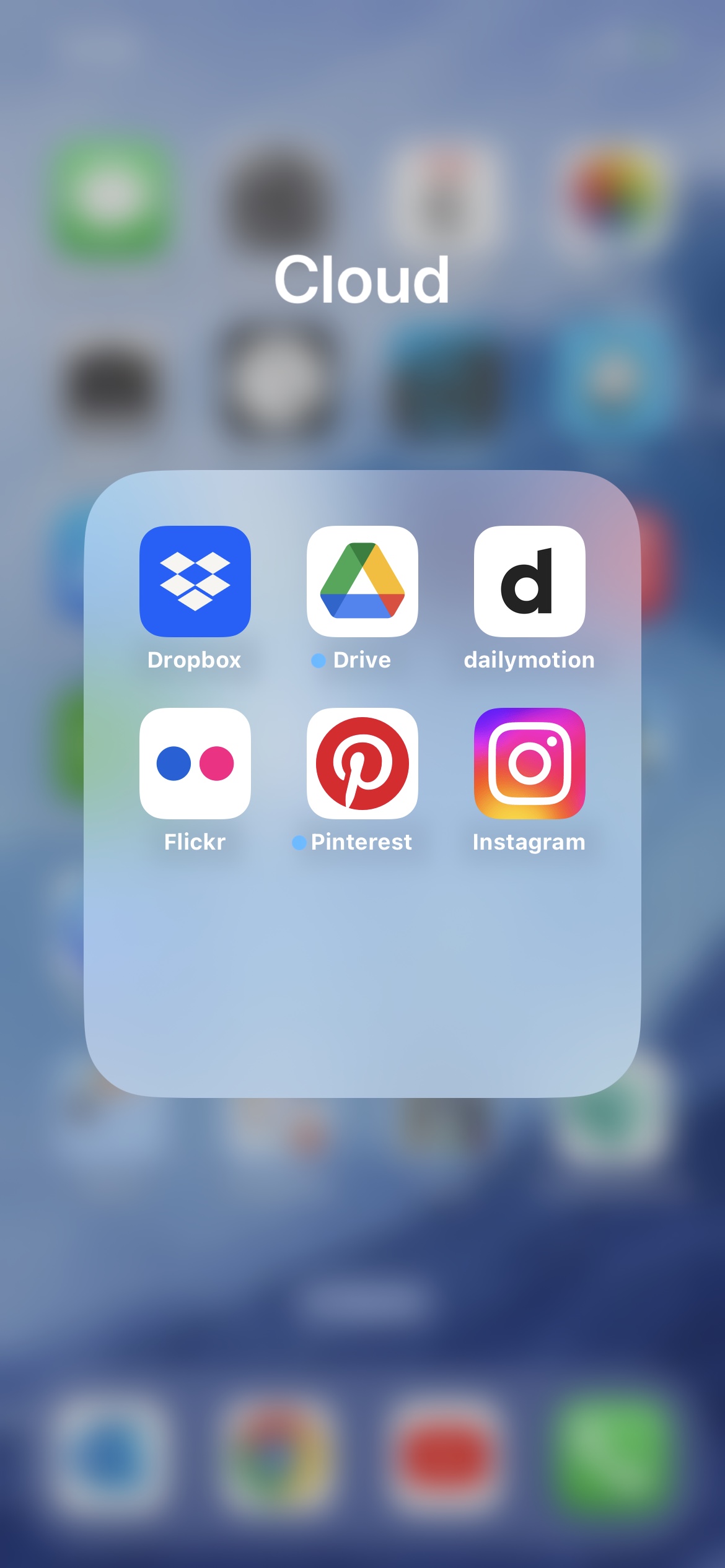The image is a detailed screenshot of a smartphone's home screen, featuring a clouded and blurred background. The screen is organized with six rows of apps, each containing four apps. Notable icons include a green messaging app in the top row and a photo app.

At the bottom of the screen, four fixed apps are visible. From left to right, these include a phone app for making calls, followed by a photos app.

In the middle of the screen, the word "cloud" is displayed prominently in white letters against a light gray square background. Within this area, several cloud-related apps are identifiable: 

- A blue app with white diamonds labeled Dropbox.
- A white app with a rainbow-colored triangle labeled Drive.
- A white app with a "D" representing Daily Motion.

On the bottom row, additional recognizable apps include:

- A blue and red dot app labeled Flickr.
- A red circle with a "P" for Pinterest.
- A rainbow-colored square with a camera icon labeled Instagram.